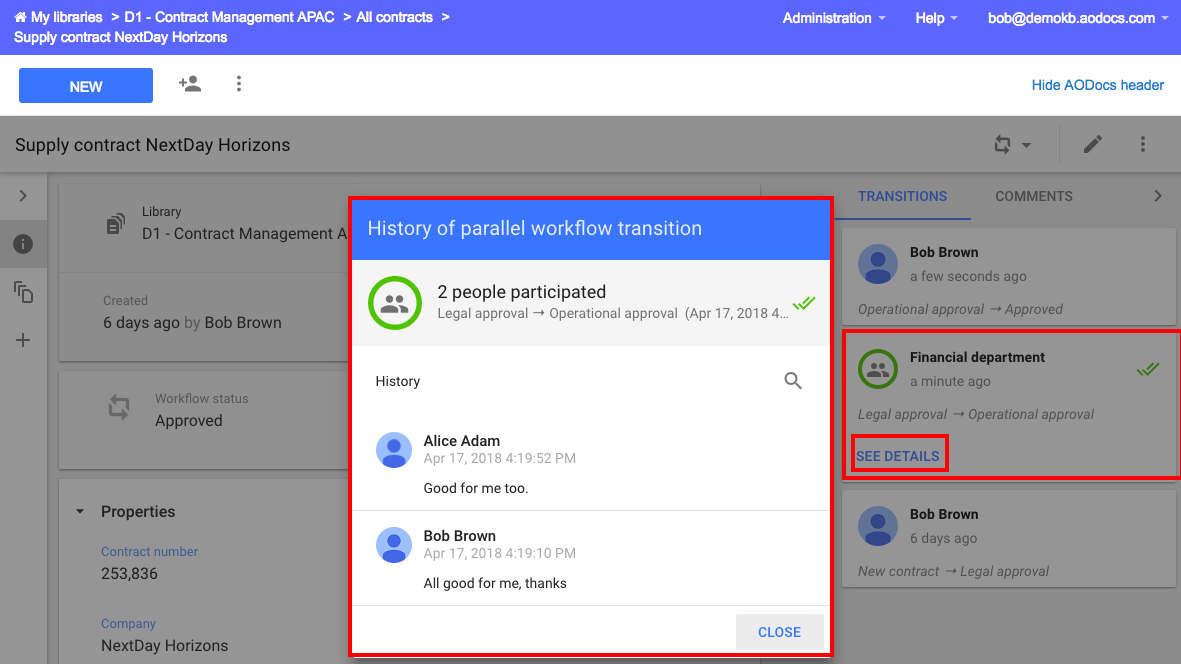The image depicts a detailed user interface of a digital contract management system. 

**Interface Layout:**
- The primary background color is white.
- On the left-hand side, there is a prominent label for managing a library of contracts named "D1."
- Below this, there is a label titled "Supply Contract Next Day Horizons" where "NextDay" is written as one word.

**Menu and Selection Options:**
- Near the top-right section, labeled "Admin help," there is a menu with dropdown options, including a contact email for support: "Bob at Dmock.adocs.com."
- Towards the center-left, within a blue box that stands out against the white background, there is a selectable option labeled "New."
- Adjacent to this, symbols include a black silhouette of a person with a plus sign and a trio of dots for additional options.

**Additional Interface Elements:**
- On the right, a blue button reads "Hide AODocs Header," whose function appears unclear.
- The gray background section beneath the white area, despite originally being written in black text, provides crucial information about "Supply Contract Next Day Horizons." This section notes that the library was created six days ago by Bob Brown and includes the contract number 256,836.

**Activity and Participation:**
- This section details transition actions taken, including:
  - Bob Brown's few seconds ago contribution.
  - An activity titled "Financial Department" recorded a minute ago.
  - Another action by Bob Brown noted six days prior.
- A pop-up features a blue bar titled "History or Play about Workflow," indicating the participation of two individuals: Alice Adams and Bob Brown, both recorded on February 17th, 2018.

This comprehensive caption effectively describes the layout, content, and navigational features of the contract management system interface as visible in the image.